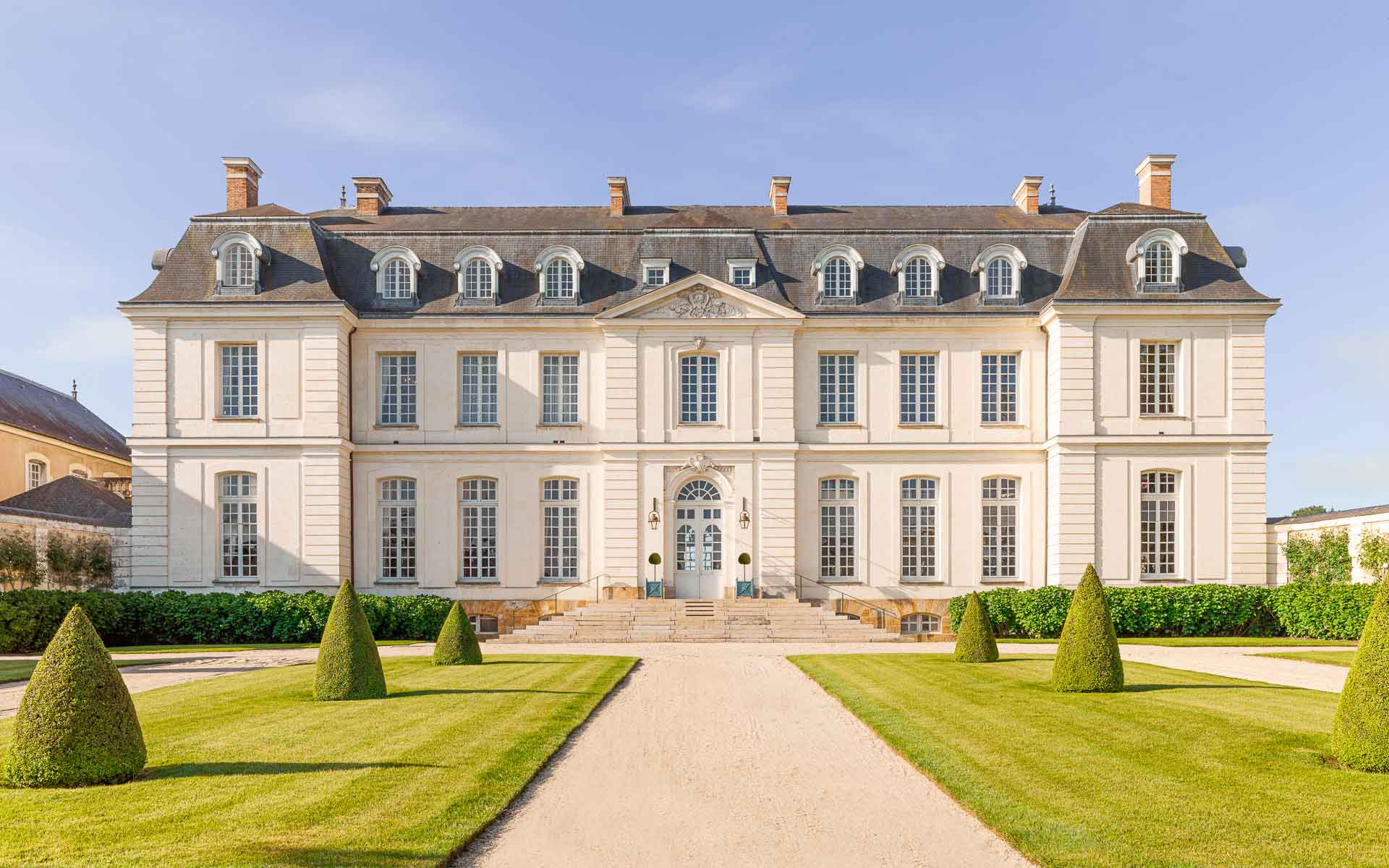This photograph captures an impressive estate, likely the home of a very wealthy individual, on a bright, sunny day with a blue sky and light, wispy clouds. The vast, cream-colored building, which spans across the image, appears to have three stories with a gray roof adorned with six red brick chimneys. The structure features distinctive white-framed windows, some of which are uniquely set into round dormer roofs. The ornate double front doors are accessed by wide, grey stone or marble steps, leading up from a long, grey pathway. The building rests atop a foundation of reddish-orange bricks. Surrounding the pathway and lawn on both sides are meticulously manicured sections of grass, featuring small triangular and cone-shaped evergreen trees, along with neatly trimmed green hedges lining the walls of the building.